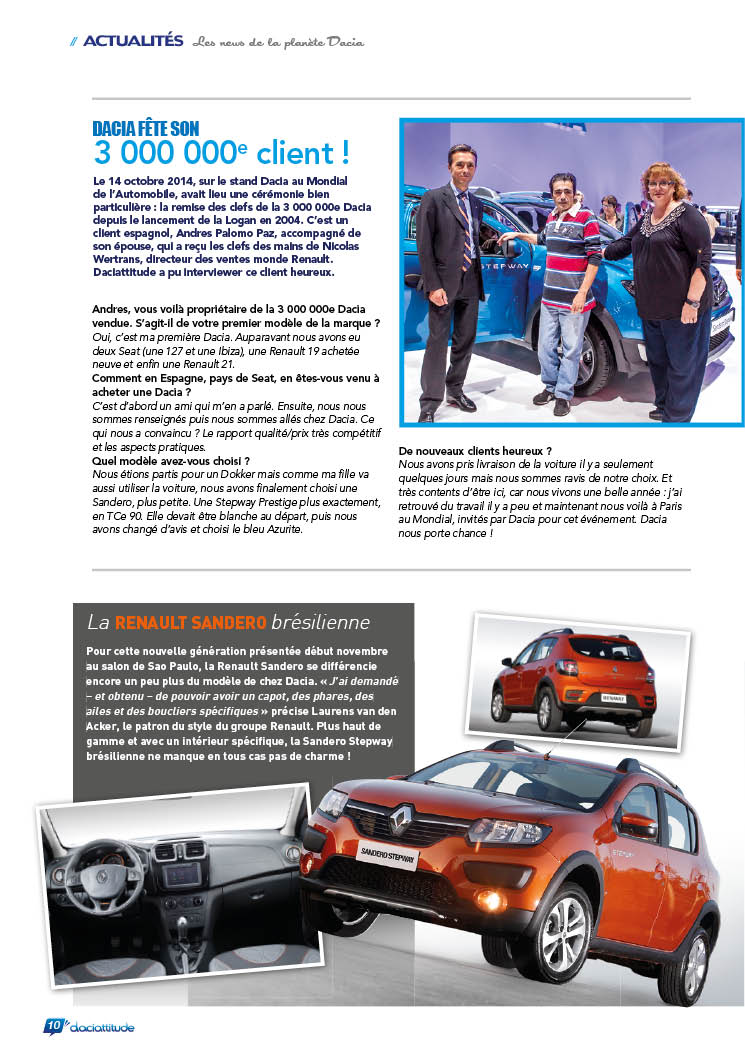The image comprises two sections of a magazine page or flyer, primarily advertising a Renault vehicle. The top half features a white background with a headline in blue text reading "Dacia Fete San, 3 Million Clients." On the right, there is a blue-bordered picture of three individuals—two men and a woman—standing next to a blue car with its doors open on a sales floor. One man is dressed in a suit, the other in a polo shirt and pants, and the woman in casual attire. Below this image, the advertisement continues with more French text.

The bottom half showcases another section of text within a grey box and features an orange Renault Sandero. The heading in this section reads "Le Renault Sandero Brasiliene" in orange font. The overall layout uses a mix of colors including black, white, several shades of blue, red, and orange, giving it a sporty and promotional appearance. The composition clearly aims to highlight the Renault Sandero with images of the car's exterior and interior, complemented by textual information primarily in French.